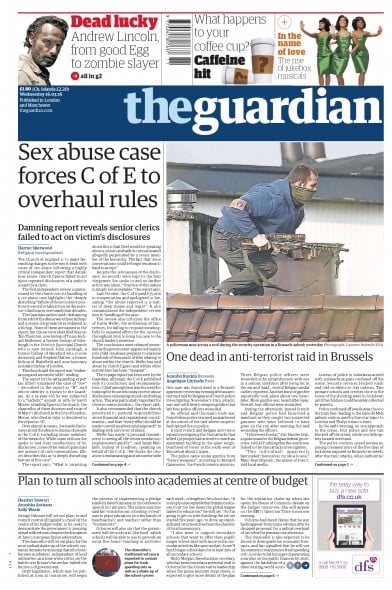Sure, here's a detailed and cleaned-up caption for the image described:

---

The front page of The Guardian features a prominent banner at the top emblazoned with "Dead Lucky" in bold, bright red text. The banner also teases an article in G2 about Andrew Lincoln, titled "From Good Egg to Zombie Slayer," though the identity of Andrew Lincoln is not elaborated upon. 

Below the banner, adjacent to the barcode area, is a subheading about coffee consumption titled "What happens to your coffee cup: Caffeine Hit." Furthermore, the phrase "In the Name of Love" hints at a piece about the rise of jukebox musicals. 

The main headlines begin with a title followed by 'PayPal or Guardian' accompanied by the publication's prices listed in the blue section typical of The Guardian's style. 

The primary headline reads "Sex Abuse Case Forces CRE to Overhaul Rules," with a subheading, "Damaging Report Reveals Senior Clerics Fail to Act on Victims' Disclosures," signaling the central news story. 

Another prominent article is accompanied by an image of a man in a khaki green balaclava, holding a firearm. The caption reads "One Dead in Anti-Terrorist Raid in Brussels," indicating significant international news.

At the bottom of the page, there's coverage on educational policy, specifically a headline stating "Plan to Turn All Schools into Academies at Centre of Budget," hinting at a major shift in the UK education system.

---

This caption provides a detailed overview of the front page, capturing all key elements and headlines accurately.